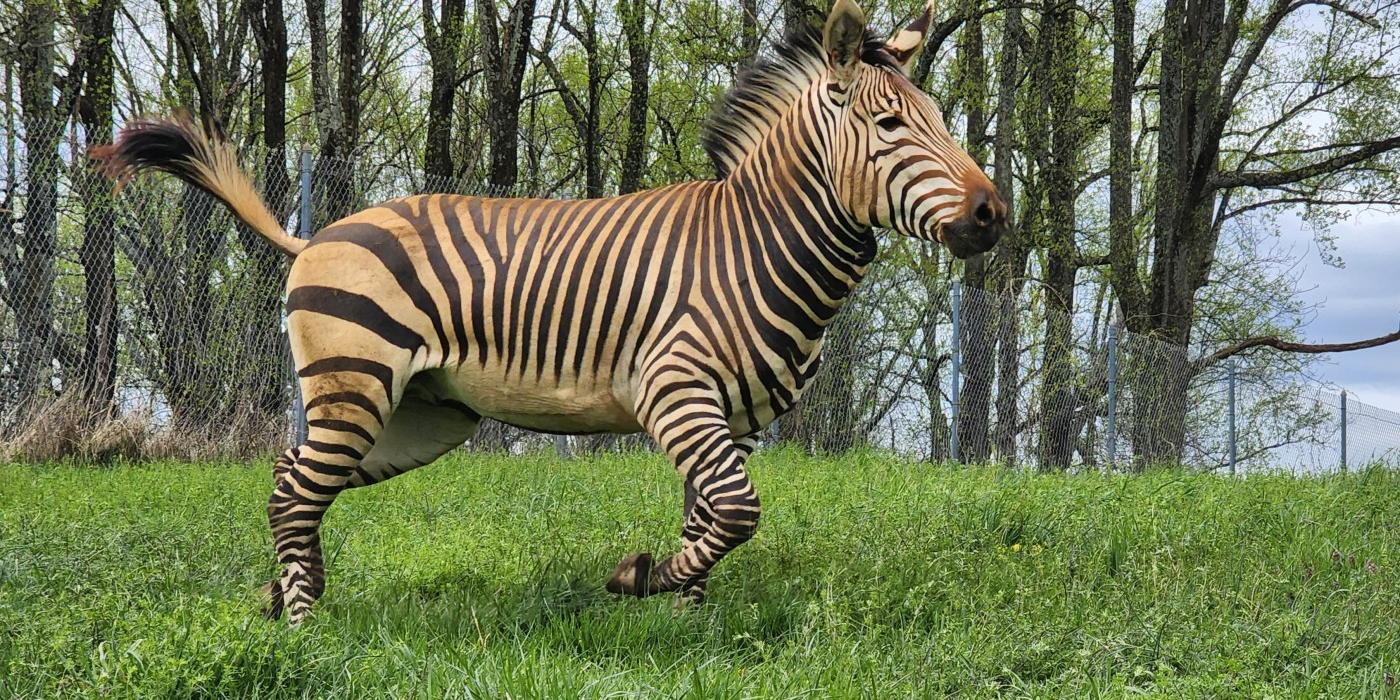This landscape image captures a dynamic scene of a zebra running across a lush green field. The zebra, covered in brown and black stripes, appears dirty, possibly from the earth beneath it. It has a distinctive white mane with black tips and black ears with white spots. The long, brown and black striped tail trails behind as it gallops from left to right, resembling the gait of a horse. Surrounding it, the verdant grass stands vibrant and healthy. Behind the zebra, a metal barbed fence with poles stretches into the distance, suggesting an enclosure. The sparse-leafed trees behind the fence contrast with the clear sky, dotted with few clouds, adding a serene backdrop to the lively scene.